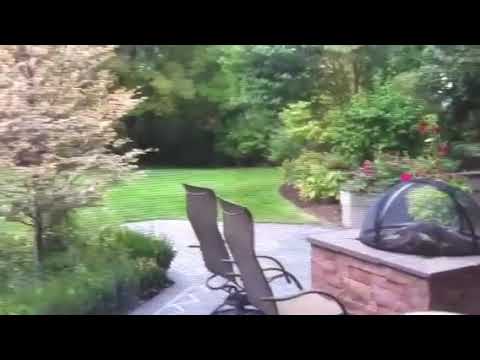The image is a slightly blurry photograph of an outdoor backyard scene bordered by black lines at the top and bottom. Dominating the foreground is a gray patio extending across the center, where a brick-based fire pit with a gray cement top and a black mesh cover is prominently placed on the right. To the left of the fire pit, there are two tan or gray chairs with long backs and dark-colored armrests, both oriented towards the fire pit. 

On the left side of the image, a tree with white flowers and a brown trunk rises above a patch of tall grass and green shrubs. Behind this area, more greenery, including a variety of bushes, small trees, and shrubs, forms a lush backdrop. The garden on the right side of the patio features a large white flower pot brimming with red or purplish flowers and vibrant green leaves. In the center of the image, the patio transitions into a light green lawn that gently curves around flowerbeds and plant areas. The entire scene is set against a cloudy sky, adding to the slightly subdued atmosphere of the outdoor space.